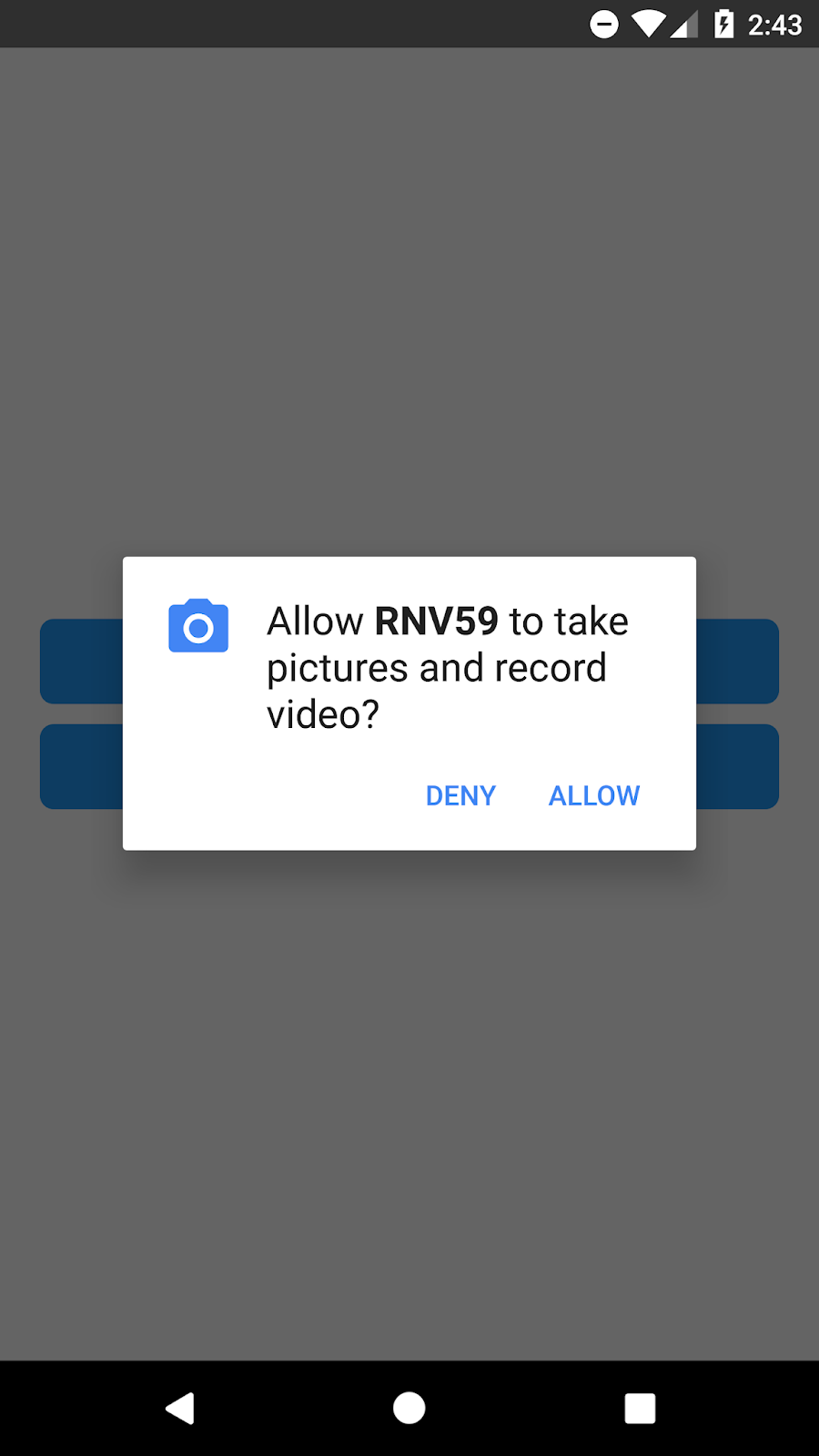The image portrays a computer screenshot with various elements present. The top section of the screen features a dark gray banner displaying partial details about the device's connectivity and status. Within this banner, the signal icon shows two out of four bars, indicating a moderate internet connection. The battery icon suggests a fully charged battery, and the time is prominently displayed as 2:43. Given the lack of additional context, it is unclear whether this indicates 2:43 AM or PM.

The majority of the screen is filled with a deep gray background. Centrally positioned on this background are two horizontal blue bars that extend across the width of the screen. These bars appear to be clickable elements or links, stacked one on top of the other. However, the content of these bars is obscured by a white pop-up window that overlaps them.

The white pop-up window, which nearly spans the entire width of the screen, has only narrow margins on both sides. A small blue camera icon is situated in the upper left corner of the pop-up. Adjacent to this icon, there is a message in bold text that reads:

```
ALLOW RNV59 TO TAKE PICTURES AND RECORD VIDEO
```

Following this, there are two interactive options at the bottom of the pop-up: "Deny" and "Allow," both presented in blue, allowing the user to choose their preferred action.